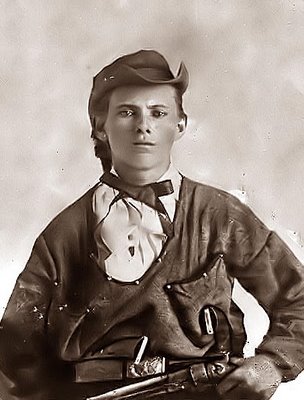This old, sepia-toned photograph features a young man captured in a traditional portrait style. The man, central in the image, gazes directly at the viewer with a composed expression. He is dressed in a white shirt layered under a black coat, and a neatly tied bow tie adorns his neck. A short hat sits atop his head, adding a touch of period authenticity. In his left hand, he holds a pistol positioned at his waist. The background blends into a light brown, sponge-textured effect, providing a muted contrast to his dark attire. Overall, his attire and the pistol suggest a historical or cowboy theme, complemented by the photo's warm brown tones.